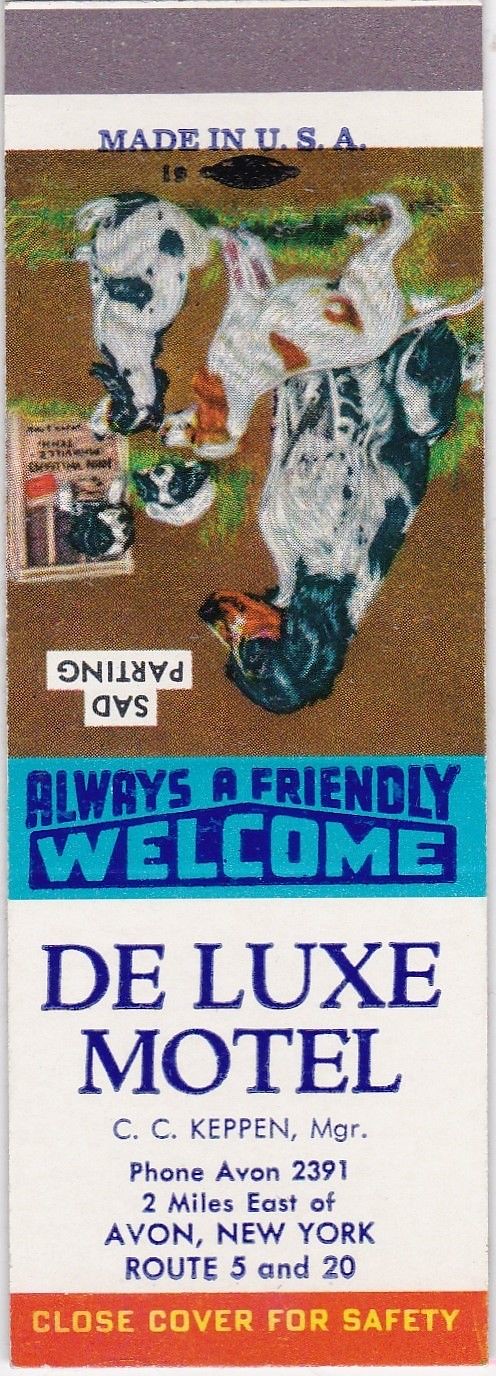The image displays a vintage matchbook with a distinct design. The top section, featuring a brownish background and a red bottom with gold text, instructs "close cover for safety." Above the red section, three illustrations of dogs are depicted, with two outside and one looking through a window, accompanied by the text "Sad Parting" - both are upside down. The words "Made in USA" appear at the top in blue. When the matchbook is flipped right-side up, the scene reorients correctly. Below the dog illustration, on a blue background with dark blue lettering, it reads "Always a Friendly Welcome." Further down, on a white background, it says "Deluxe Motel," followed by "C.C. Keppen, Manager (MGR)" in blue text, and the phrase "Phone: AVON 2391, 2 miles east of AVON, New York, Route 5 and 20." The matchbook's text emphasizes the classic safety reminder: "close cover for safety."